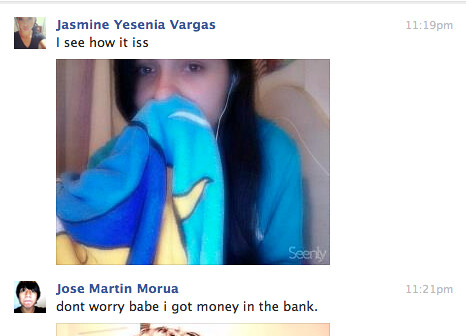The screenshot captures a Facebook post from Jasmine Yesenia Vargas at 11:19 PM, stating "I see how it is," followed by an image of herself. In the photo, Jasmine has long black hair and is wearing a dark tank top or V-neck shirt and light blue pajamas. She is holding a brightly colored towel, possibly with a Disney theme, up to her mouth, and wears corded earbud headphones while looking at the camera. Her post is followed by a comment from Jose Martin Morua at 11:21 PM, saying, "Don't worry, babe, I got money in the bank." The comment thread appears on a white background, and a portion of a second image is partially cut off at the bottom of the frame.